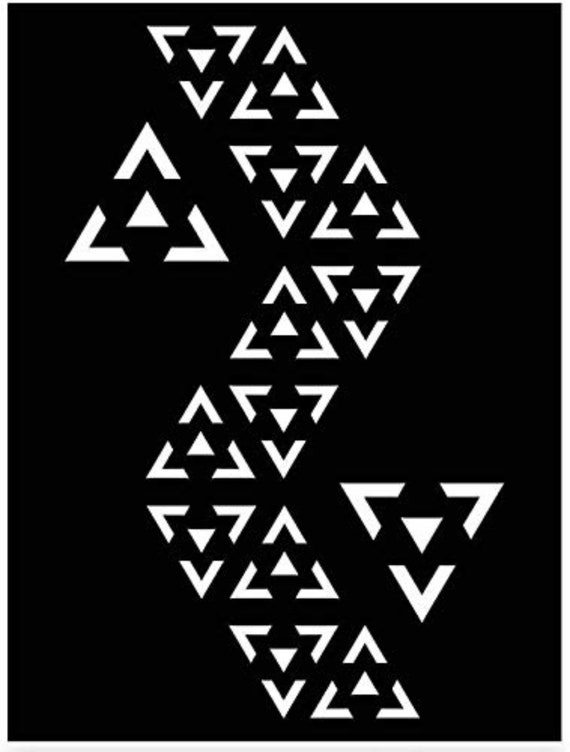This image features a striking design set against a solid black background, showcasing a complex arrangement of white and black triangles. Dominating the design are two large triangles: one on the left pointing upwards, and one on the right pointing downwards. These triangles are part of a repetitive three-layer pattern, where each large white triangle contains a smaller, inverted black triangle, which is further layered with an even smaller white triangle. This intricate pattern forms a continuous sequence, zigzagging diagonally across the center of the image. The zigzag starts from the middle top, moves down to the right, shifts to the left, and then heads back to the right, creating a dynamic line of intersecting triangles. In total, there are four turns in the zigzag, with each turn comprising these layered, alternating triangles. The overall effect is a mesmerizing, geometric tapestry that combines symmetry, contrast, and movement.